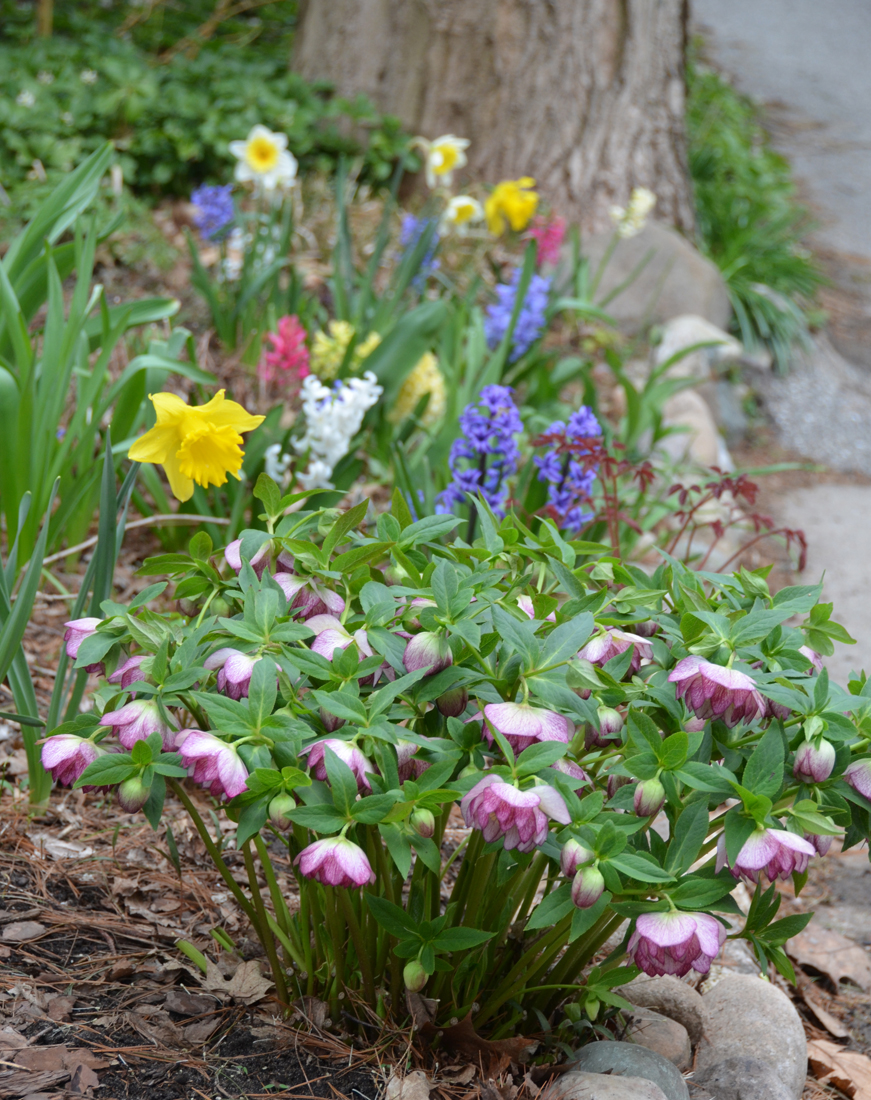The photograph displays a vibrant array of flowers along a sidewalk, capturing a rich mix of colors and floral varieties. In the foreground, there are dark pink and white flowers with petals that droop down from their stems, surrounded by numerous green leaves. Adjacent to these, on the left, is a bright yellow daffodil, also on a green stem. Behind these flowers, there is a collection of yellow daffodils, purple, white, and pink flowers that resemble hyacinths or lilacs, and additional white and yellow daffodils. The background reveals the lower part of a tree trunk, with surrounding green bushes, grass, and pine straw. The right side of the image features stone edging for the flower bed, leading to a cracked concrete sidewalk or stone walkway. The variety of flowers, including mentions of an Indian brush and bluebonnets, adds to the picturesque garden scene, which is framed by natural and built elements, lending a structured yet lush ambiance to the photograph.